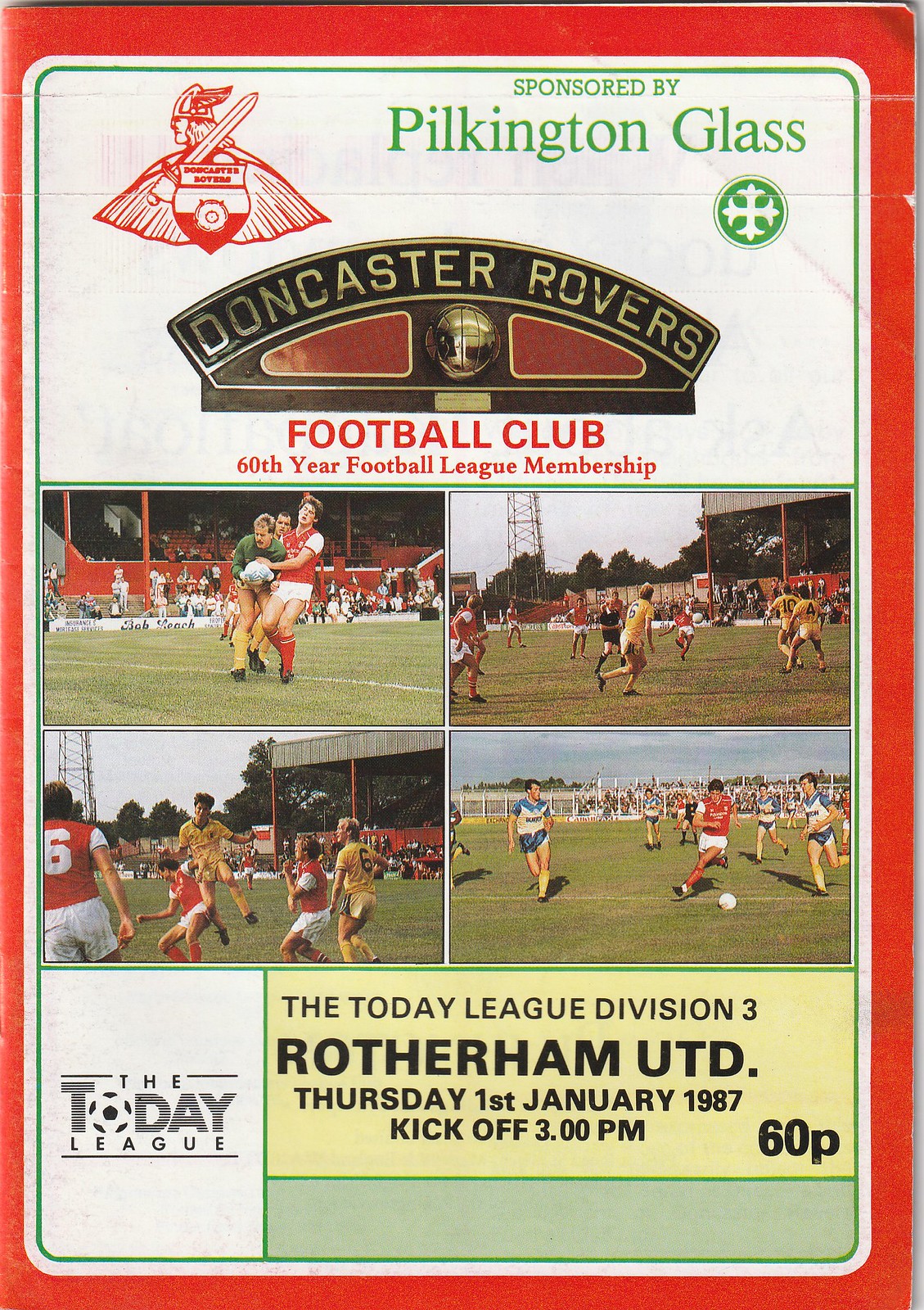The image depicts the cover of a sports program or magazine, prominently featuring a red border framing the entire picture. At the top left is the Doncaster Rovers Football Club logo, which illustrates a Viking holding a sword over his shoulder and a shield, with sponsorship from Pilkington Glass in green text. This program commemorates Doncaster Rovers' 60th year of football league membership. The background is primarily white, and the cover includes four separate photographs of soccer players in action, all taken outdoors during the daytime. Audience members can be spotted to varying degrees in these photographs, suggesting they were taken at different locations. The bottom of the cover provides specific event details: "Today League Division III, Rotherham United, Thursday, 1st January 1987, kickoff at 3pm," with an admission cost of 60p displayed in the lower right corner.